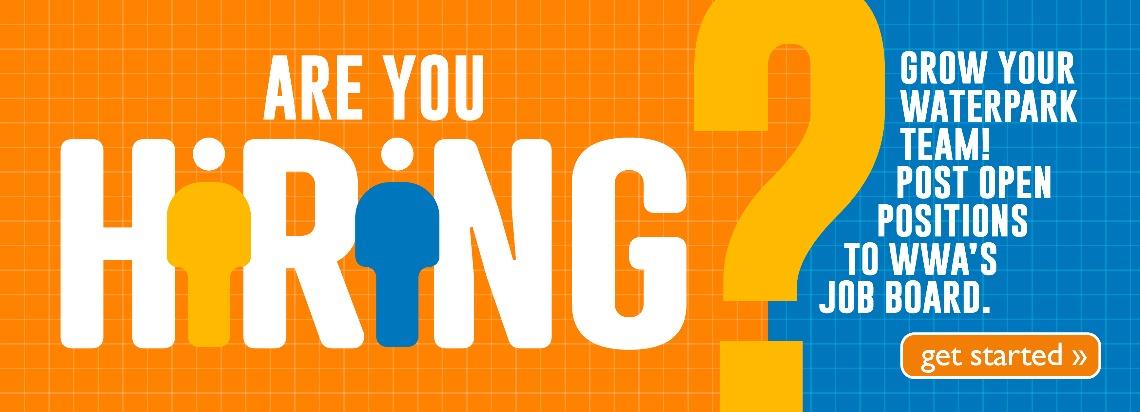This image is a banner advertisement from an unknown website designed to attract employers seeking to expand their water park teams. The banner is significantly wider than it is tall and features a split background. The left side showcases a bright orange background with the text "Are you hiring?" written in bold, white letters. The two "I"s in "hiring" are stylized to resemble people, with the first "I" colored orange and the second "I" in blue, followed by an orange question mark. 

The right side of the banner has a blue background and includes the text, "Grow your water park team. Post open positions to WWA’s job board." At the bottom right corner, there is an orange oblong button that says "Get Started" in white letters, accompanied by two white arrows pointing to the right. The banner is minimalist, featuring no people, animals, birds, plants, buildings, automobiles, airplanes, boats, mountains, or bridges.